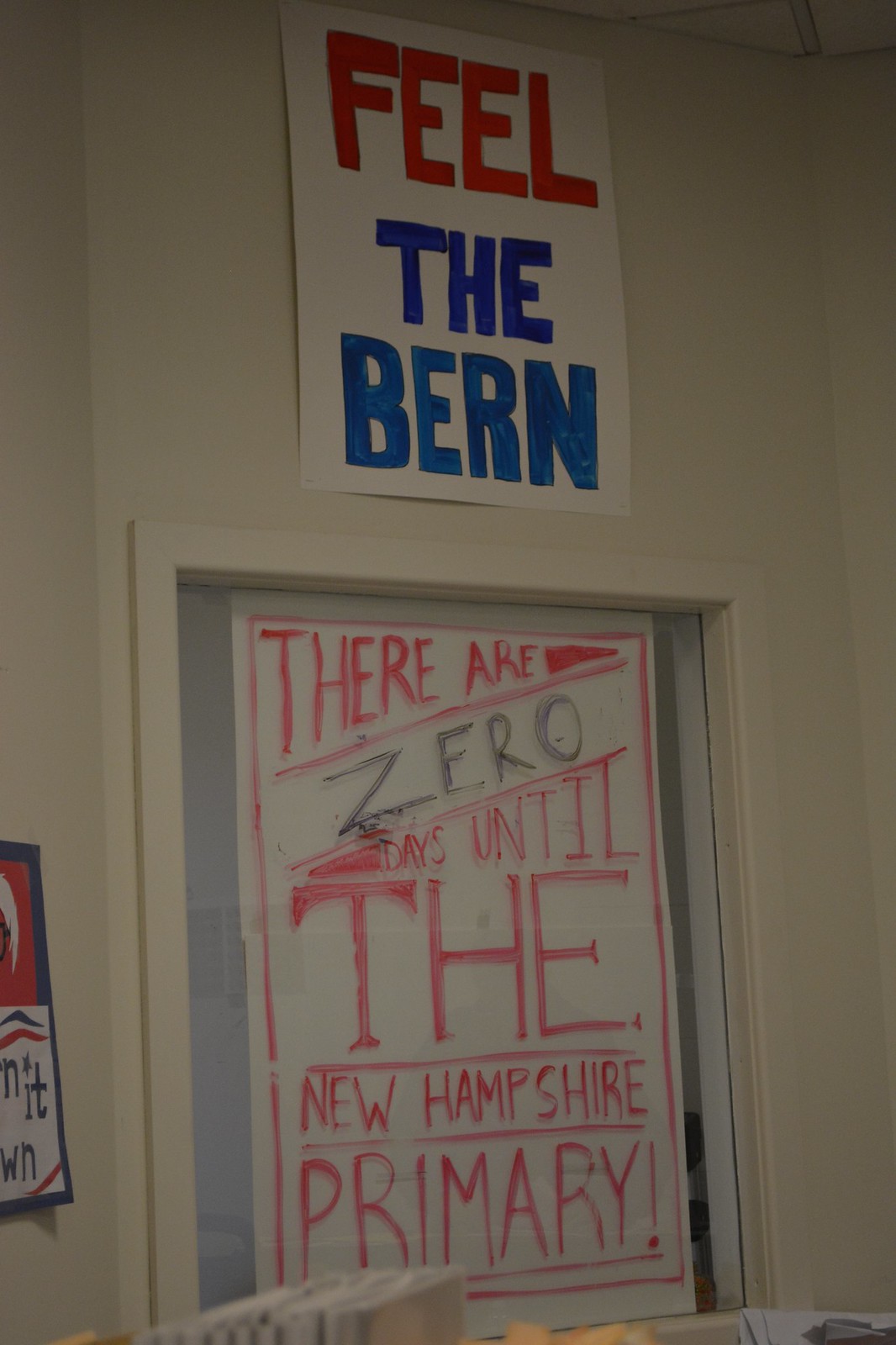In this image, we see a scene of political campaigning likely for the New Hampshire primary. The setting is an indoor space with featureless beige walls. A large window, which dominates the lower part of the image, is covered by a prominent handmade white poster. This poster has a red border and bold text stating, "There are zero days until the New Hampshire primary," with the word "zero" emphasized in black while the rest of the text is in red. Above this window hangs another white poster, urging viewers to "Feel the Bern" in support of Bernie Sanders. The phrase "Feel" is highlighted in red, while "Bern" is accented in blue, spelling "Bern" as B-E-R-N to reference Sanders. The handmade nature of the signs, with their colorful and contrasting fonts, draws attention and underscores the urgency and grassroots enthusiasm of the campaign.